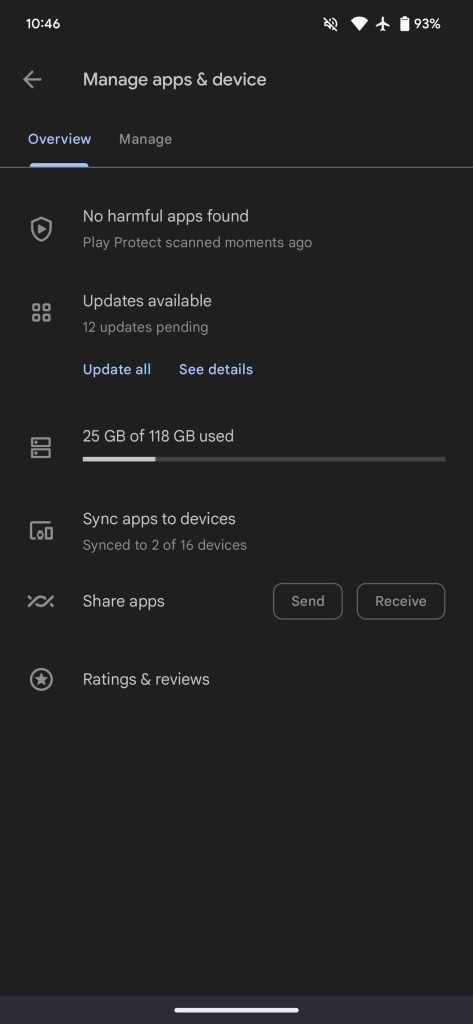The image displays a screenshot from a website, captured on a cell phone. The background is entirely black. At the top of the screen, white text indicates the time: "10:46". To the right, there is an icon of a speaker with a diagonal line through it, indicating it is muted. Next to it, various icons provide information: a Wi-Fi symbol, an airplane mode icon, and a battery icon showing "93%".

Below this, a left arrow icon is shown, beside which is the text "Manage apps & devices" with a capital 'M'. Directly underneath, the word "Overview" is displayed in a bluish-white, underlined font. Below this are more details in the same bluish-white font, including:

- "No harmful apps found, Play Protect scanned moments ago."
- "Updates available, 12 updates pending. Update all | See details."
- "25 GB of 118 GB used," accompanied by a progress bar showing usage.
- "Sync apps to devices," indicating "Synced to 2 of 16 devices."
- "Share apps," alongside options to "Send" or "Receive" in white text with a white border.

Lastly, the section "Ratings and reviews" is displayed at the bottom.